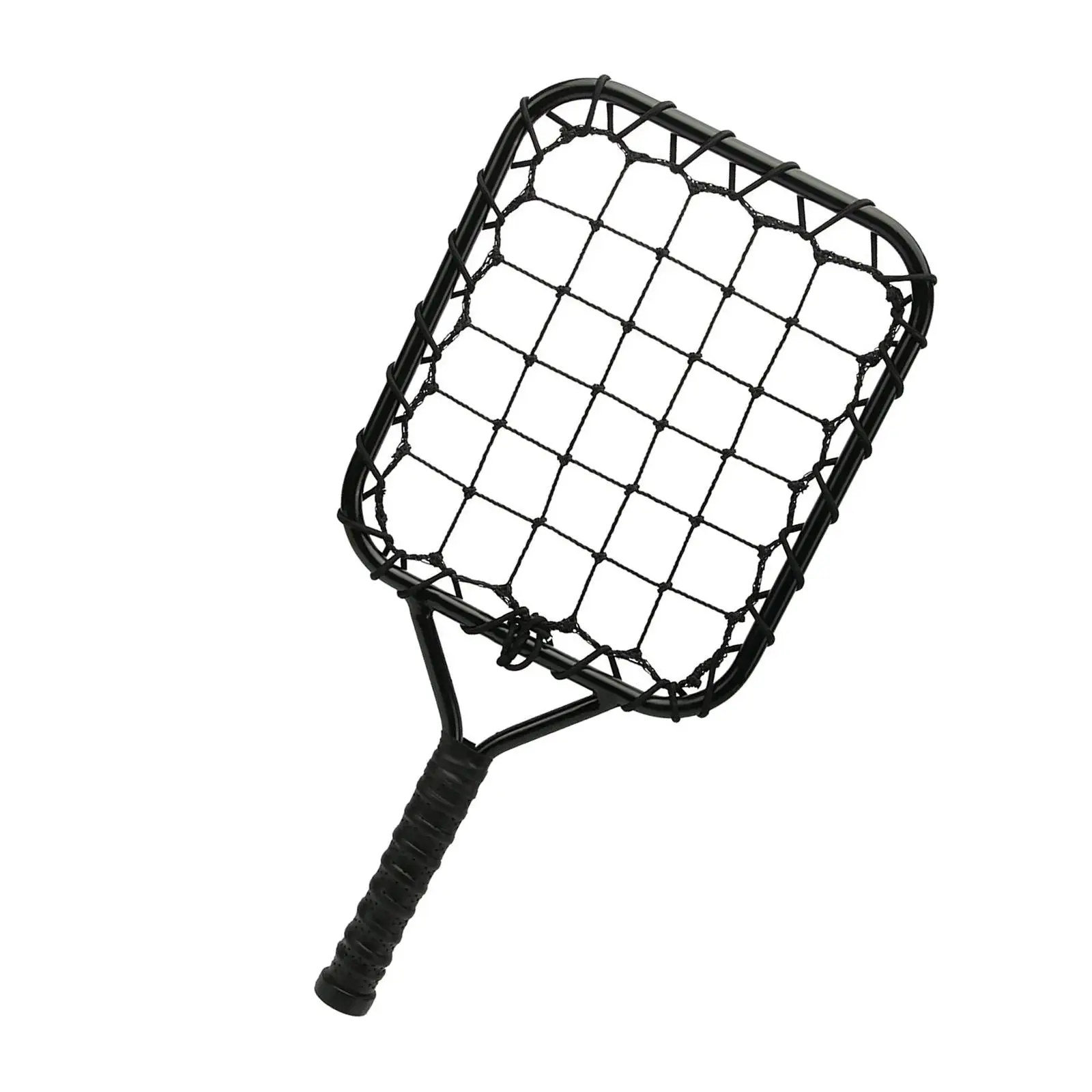This photograph captures a unique piece of sporting equipment. The racket prominently features a sturdy black metal frame with a short handle wrapped in a black grip, likely rubber or tape. The handle is positioned towards the bottom left of the image, extending diagonally to the top right where the net is situated. The net itself is composed of thick, nylon strings woven into large squares, forming a grid-like pattern that's distinctively spacious compared to typical tennis rackets. The net structure is rectangular yet rounded at the edges, creating a less traditional shape that hints at its use in a specialized, possibly outdoor, sport. The lack of a background or border emphasizes the simplicity and focus on the racket's unique design.